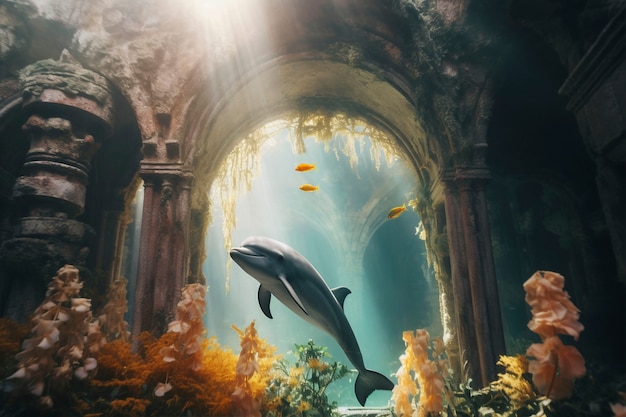The painting depicts a serene underwater scene centered around a graceful dolphin swimming within a ruined underwater palace. The palace, constructed of weathered brownish stone, features tall pillars and magnificent arched doorways that hint at its former grandeur. Now, the structure is overrun with colorful marine life, including vibrant orange and yellow corals that resemble underwater flowers, and various algae with petal-like growths. 

Light penetrates the water from above, illuminating the scene and adding a mystical glow that highlights the high ceilings and intricate architecture. The dolphin, predominantly gray with a lighter underside, is captured in a moment of elegance, moving towards the upper left through one of the grand archways. Surrounding it are several small golden fish, adding to the lively ambiance of the picture.

A prominent circular column, reminiscent of a totem pole, stands next to the left pillar, while plant growths adorn the upper sections of the walls, indicating the pervasive nature of sea life. The overall composition beautifully merges the tranquility of the underwater world with the haunting beauty of a lost, submerged civilization.